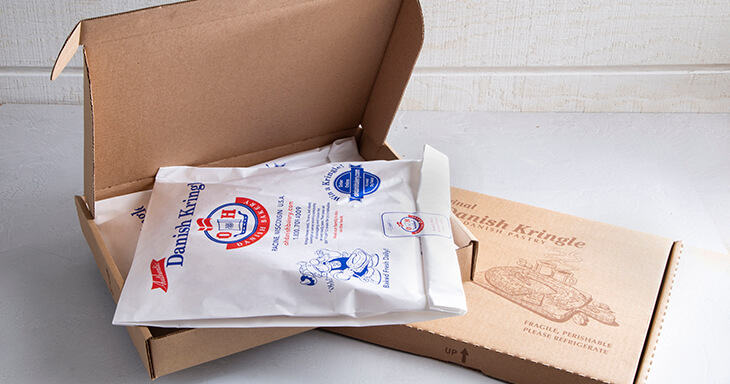This detailed photograph, taken indoors against a white counter and a white wall, captures two cardboard boxes of Danish Kringle pastries, emphasizing their perishable nature. The open box reveals a sealed white pouch emblazoned with "Danish Kringle" and "Racine, Wisconsin." The pouch features a decorative emblem with the letters "OH" and a central symbol. To the lower left of the pouch, a Viking graphic depicts a figure holding bread with "Baked Fresh Daily" underneath, while to the right sits a blue emblem stating "Win A Kringle." Adjacent to this box is a closed cardboard box with labels reading "Danish Kringle," "Danish Pastry," "Fragile," "Perishable," and "Please Refrigerate," as well as a graphic illustration of the Kringle bread. The photograph's subtle shading adds depth, highlighting the contents and instructions on each box, underscoring the delicacy and care required for these pastries.